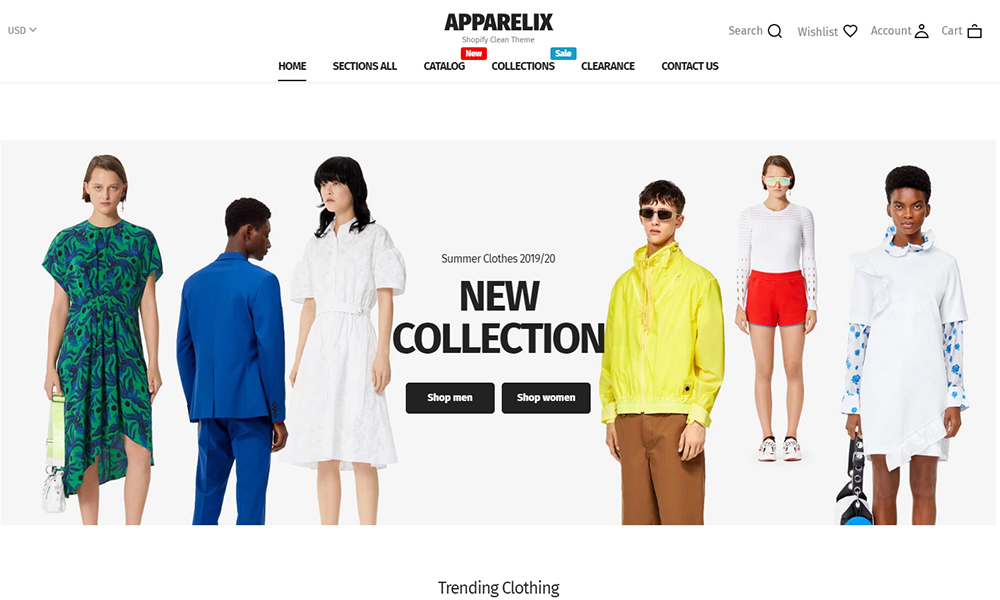The front page of the clothing website "Apparelix" is designed with a clean, white background. Located in the upper left corner is "USD" in gray text, accompanied by an arrow that likely allows users to change the pricing currency. At the center top, the site's name, "APPARELIX," is prominently displayed in bold, black capital letters. Featuring at the far right are icons for different functionalities: a magnifying glass for search, a heart for the wish list, a silhouette for the account, and a briefcase representing the shopping cart.

Beneath the site title, there is a line of gray text that appears to read "Shopify clean theme," though it is somewhat difficult to decipher. Below this, several navigation options are available, displayed horizontally: "Home" (currently selected), "Sections All," "Catalog" (highlighted with a red square and white text indicating "new"), "Collections" (marked by a blue square with white text reading "sale"), "Clearance," and "Contact Us."

Following the navigation menu is a prominent image with a light gray background, showcasing several models in various clothing items. From left to right:

1. A Caucasian female with short brown hair wearing a blue-green dress that resembles peacock feathers. She is accessorized with a white bag with a light green strap.
2. A black male facing away from the viewer, showcasing a blue suit with a visible jacket and pants.
3. A female, possibly of Asian descent, with long dark hair wearing a white short-sleeved dress.

Centered within this image is the text "Summer Clothes 2019-20, New Collection," alongside two black buttons with white text: "Shop Men" and "Shop Women."

Continuing further:

4. A male with short brunette hair, clean-shaven, wearing sunglasses, a gray windbreaker jacket, and brown pants.
5. Another female, seemingly the same model as the first one on the far left, in a white long-sleeved shirt with cutouts or squares on the forearms, orange shorts, sneakers, and neon-colored glasses.
6. A female with shortly cropped hair in a long white t-shirt layered over a long-sleeved shirt featuring blue designs. She holds a white bag with black trim, blue sides, and a black strap adorned with silver metal holes.

At the bottom of the page, "Trending Clothing" is spelled out in black text, with both "Trending" and "Clothing" starting with capital letters.